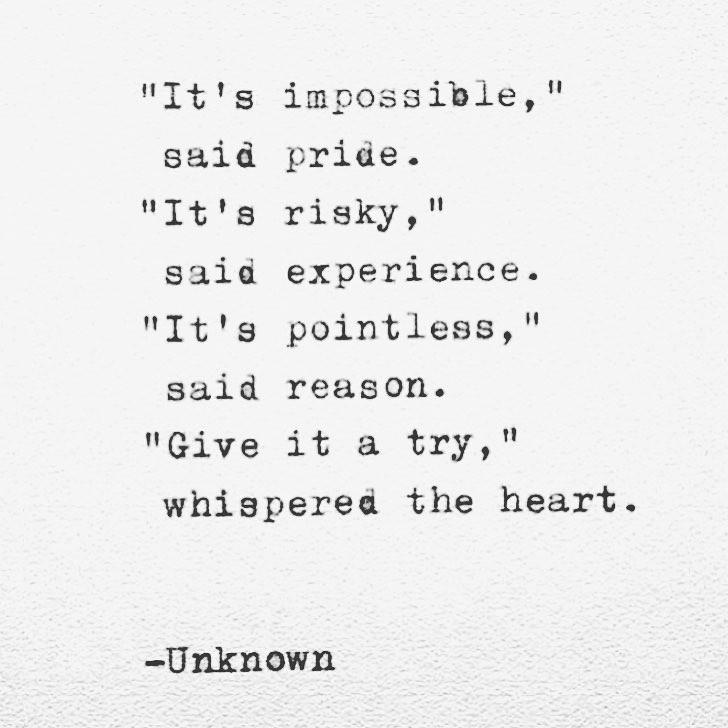The image displays a set of quotes formatted to resemble a poem, positioned on a textured, off-white or parchment-like background that evokes the feel of handmade or heavy stock paper. The text is presented in a typewriter font, suggesting either a vintage typewriter or a digitally replicated typewriter style. The quotes read: "It's impossible," said pride. "It's risky," said experience. "It's pointless," said reason. "Give it a try," whispered the heart. Beneath these lines, the word "unknown" is inscribed, signifying the author's anonymity. The text is centrally aligned, occupying the middle of the image both vertically and horizontally, creating a balanced and visually appealing composition. Some parts of the text show slight fading, enhancing the nostalgic and aged aesthetic.